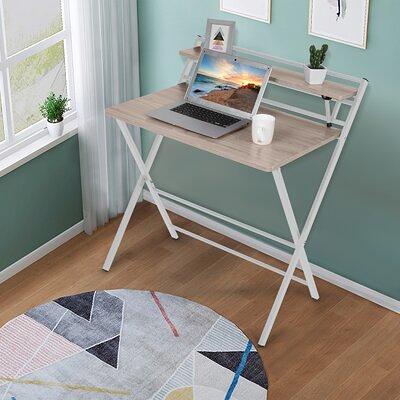The image displays an immaculately clean room with walls painted in a calming aqua green. Against these walls stands a small computer desk, characterized by its white metal legs and light brown wooden surfaces. The desk, complete with a single upper shelf, fits snugly beneath two picture frames that contain simplistic white designs. Adjacent to the desk is a window, partially visible, with crisp white trim and white curtains. The window sill supports a small plant in a white pot. The floor is a light hardwood, subtly complemented by an abstract, circular rug featuring a collage of shapes and colors including gray, black, red, yellow, and blue. On the desk, a laptop displaying a scenic beach background is placed alongside a white mug and a candle. On the shelf above, there is a small picture frame and another white pot housing a cactus, enhancing the serene and meticulously arranged aesthetic of the space. The overall layout and lighting of the scene give it a digitally rendered appearance, with some elements appearing disproportionate and possibly inserted via computer.